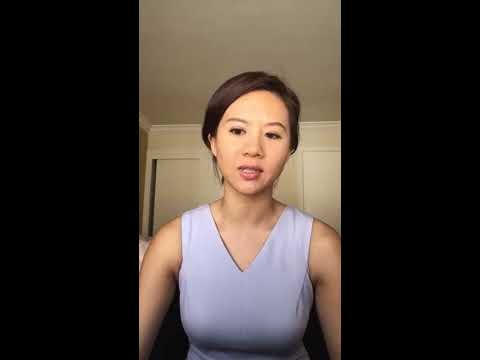This image appears to be a screenshot of an unhappy-looking Asian woman participating in a video chat, perhaps via FaceTime or another similar platform, which is indicated by the black borders on the left and right sides of the frame. The woman, wearing a sleeveless, V-neck, tight lilac dress that highlights her well-defined shoulders and arms, is captured from the torso upwards. Her black hair is neatly tied back in a bun, and her lips are accentuated with pink lip gloss or lipstick. Her expression is one of shock or displeasure, suggesting she may have been unaware of the photo being taken or is unhappy with how she appears. The background shows beige or cream-colored walls of an apartment, with little to no decor visible, focusing the viewer's attention on the woman. Additionally, the image hints at other architectural features like doors, potentially to a closet or bathroom. She appears to be seated, evidenced by the subtle light reflections on her face and arms, likely from a lamp. Her slightly open mouth suggests she might be in the midst of speaking.